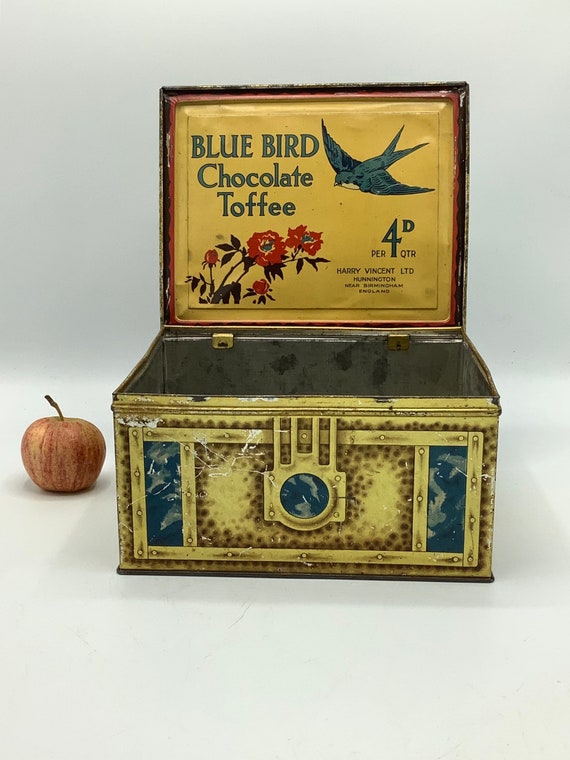This image depicts an antique metal tin box, possibly dating from the 1890s to 1920s, designed to resemble a treasure chest with teal and fake gold accents. The tin's lid is open, revealing a gray metal interior. Inside the lid, "Blue Bird Chocolate Toffee" is written in blue blocky letters, accompanied by an image of a blue bird in mid-flight above red flowers with green stems and leaves. The inscription also reads, "P.E.R. 4D Q.T.R. per 4D quarter," and mentions "Harry Vincent Limited, Harrington something, Birmingham, England." To the left of the tin, there is an apple with a subdued red color, placed against a plain white background to provide scale. The tin itself also features an image of the front of a chest with a blue colored lock, and one of the brackets that would keep the tin together is visible.